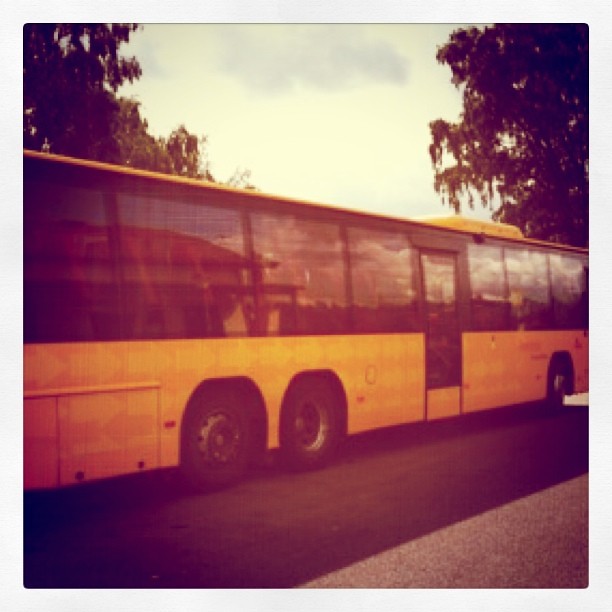The photograph depicts a vintage, elongated bus with desaturated colors, giving the image an aged appearance reminiscent of the 1950s or 1960s. The bus, primarily shown from a side profile, has a rectangular shape without a protruding engine section. Its lower half appears yellow, likely due to color desaturation, while the upper section features large, square, black-tinted windows that reflect the sky and surrounding environment, preventing any view of the bus's interior. Notably, the bus has a prominent door positioned after three windows, along with lower compartments likely meant for luggage. There are three visible black wheel wells and wheels. Arrow decals point toward the front of the bus, enhancing its streamlined look. The scene above the bus includes overhanging trees on both sides, which seem dark green due to the image’s color editing, and a sky filled with muted blue clouds. The bus casts a shadow on the black asphalt road it stands on, completing the nostalgic snapshot with a touch of vintage charm.